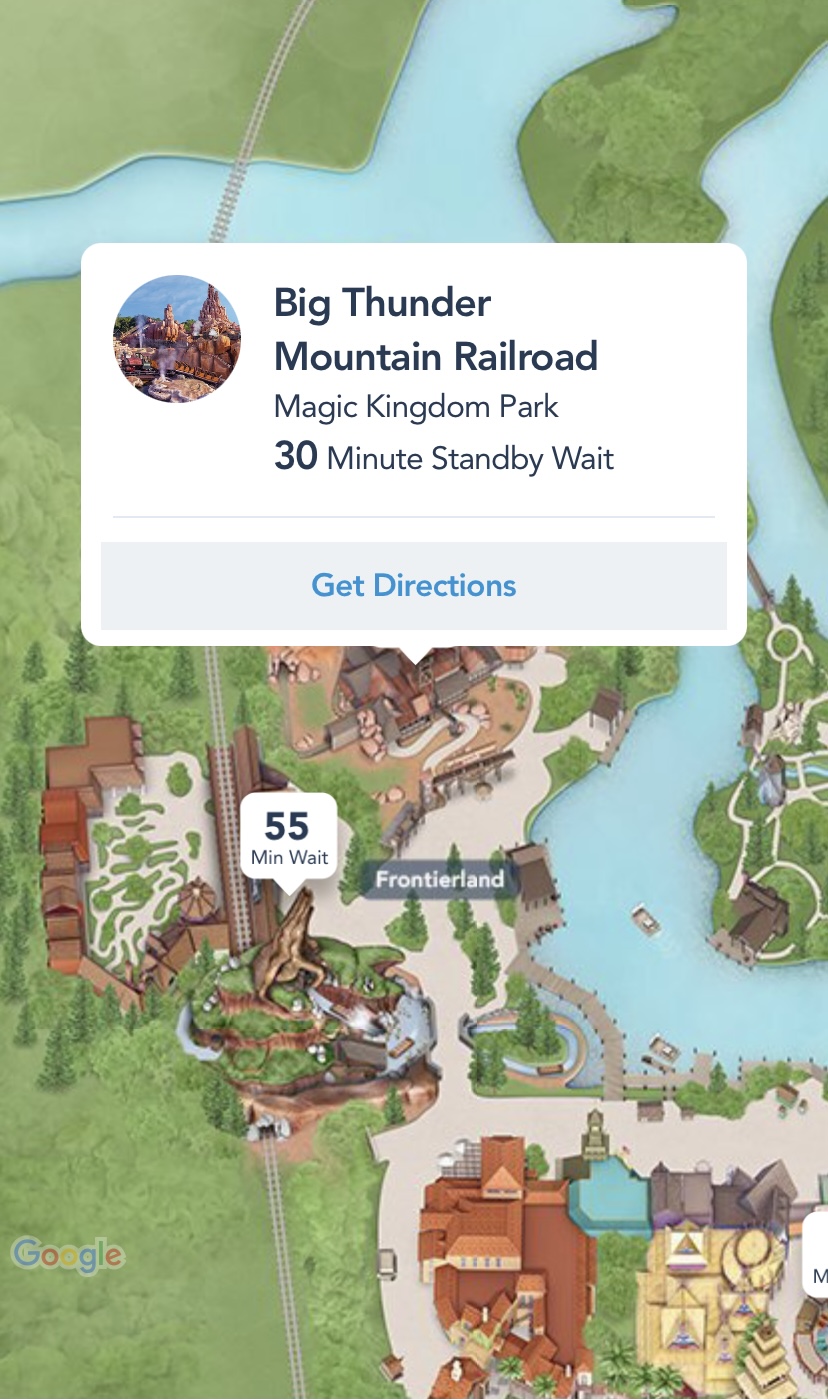This is a detailed screenshot of a Google Maps page displaying a theme park, which visually resembles a game map with stylized graphics. Prominently, a pop-up window is positioned near the top of the image. This window features a white background and contains the title "Big Thunder Mountain Railroad" in bold black letters. Beneath the title is the location "Magic Kingdom Park," followed by information stating a "30 minute standby wait." Below this, there is a gray 'Get Directions' button highlighted with blue text. To the left of the text, there is a circular image depicting the location. The map itself showcases a park layout with notable bodies of water resembling rivers, and various attractions and facilities situated along the waterfront.